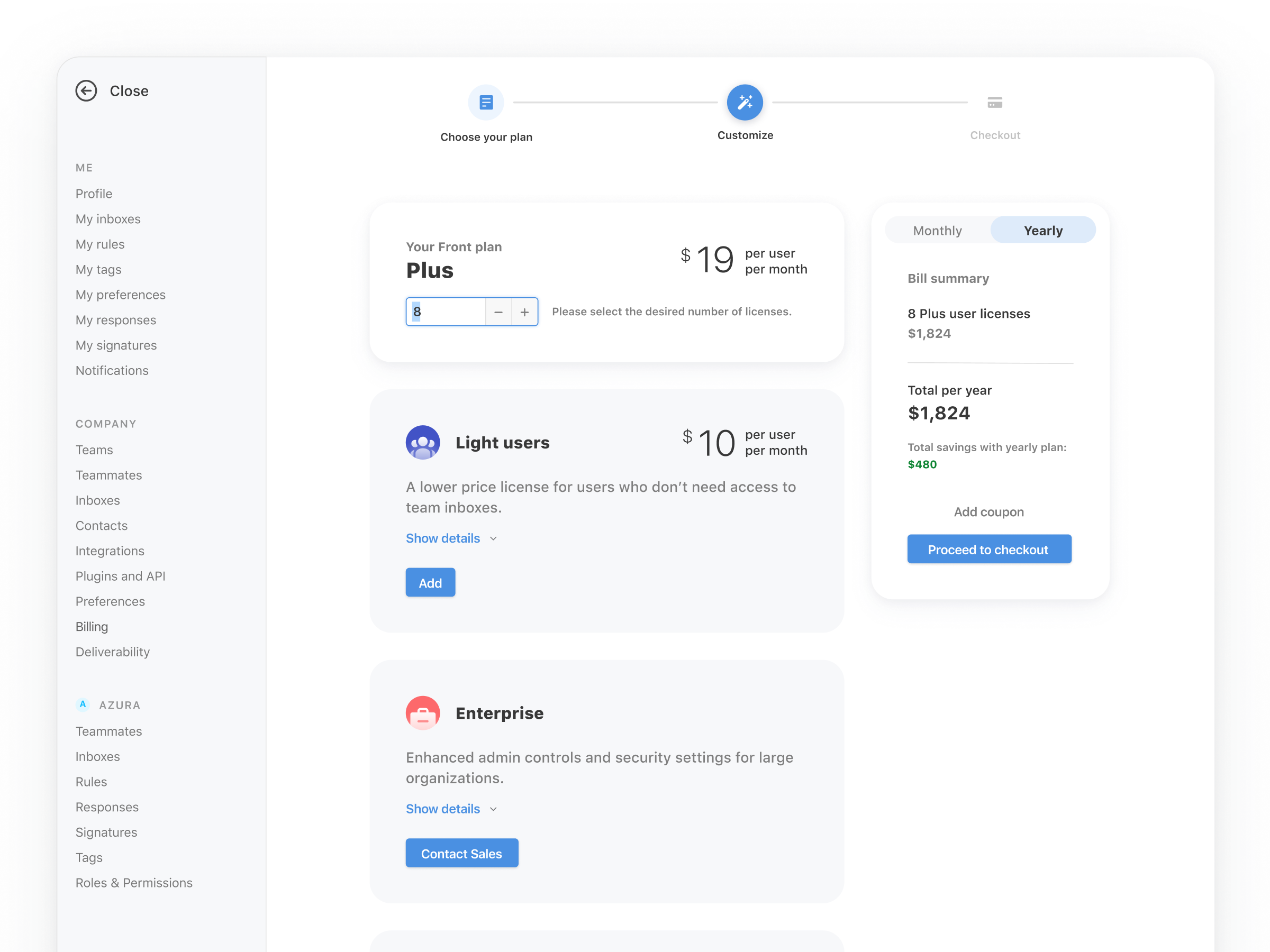This image is a screenshot of a webpage displaying a pricing and plan selection interface. At the top of the page, the heading reads "Choose Your Plan," followed by a navigational path indicating the steps: "Customize" (illustrated with a magic wand icon inside a blue circle) and "Checkout."

Beneath this navigation, the various plan options are outlined:

- **Plus Plan**: This plan costs $19 per user per month. In this instance, the user has selected 8 licenses. There is a prompt to "Please select the desired number of licenses."
- **Light Users Plan**: Priced at $10 per user per month, this option is for users who do not need access to team inboxes.
- **Enterprise Plan**: This plan offers enhanced admin controls and security settings tailored for large organizations.

To the right of these options, there is a toggle for selecting "Monthly" or "Yearly" billing. The user has chosen the "Yearly" option.

Below the plan details, a summary of the billing details is provided:
- **8 Plus user licenses**: totaling **$1,824 per year**.
- The "Total Savings with Yearly Plan" is highlighted in green, showing a savings of **$480**.
- There is an option to "Add Coupon" and a button to "Proceed to Checkout."

This detailed page guide leads the user through selecting and customizing their desired plan, clearly displaying the costs and savings associated with the yearly billing option.